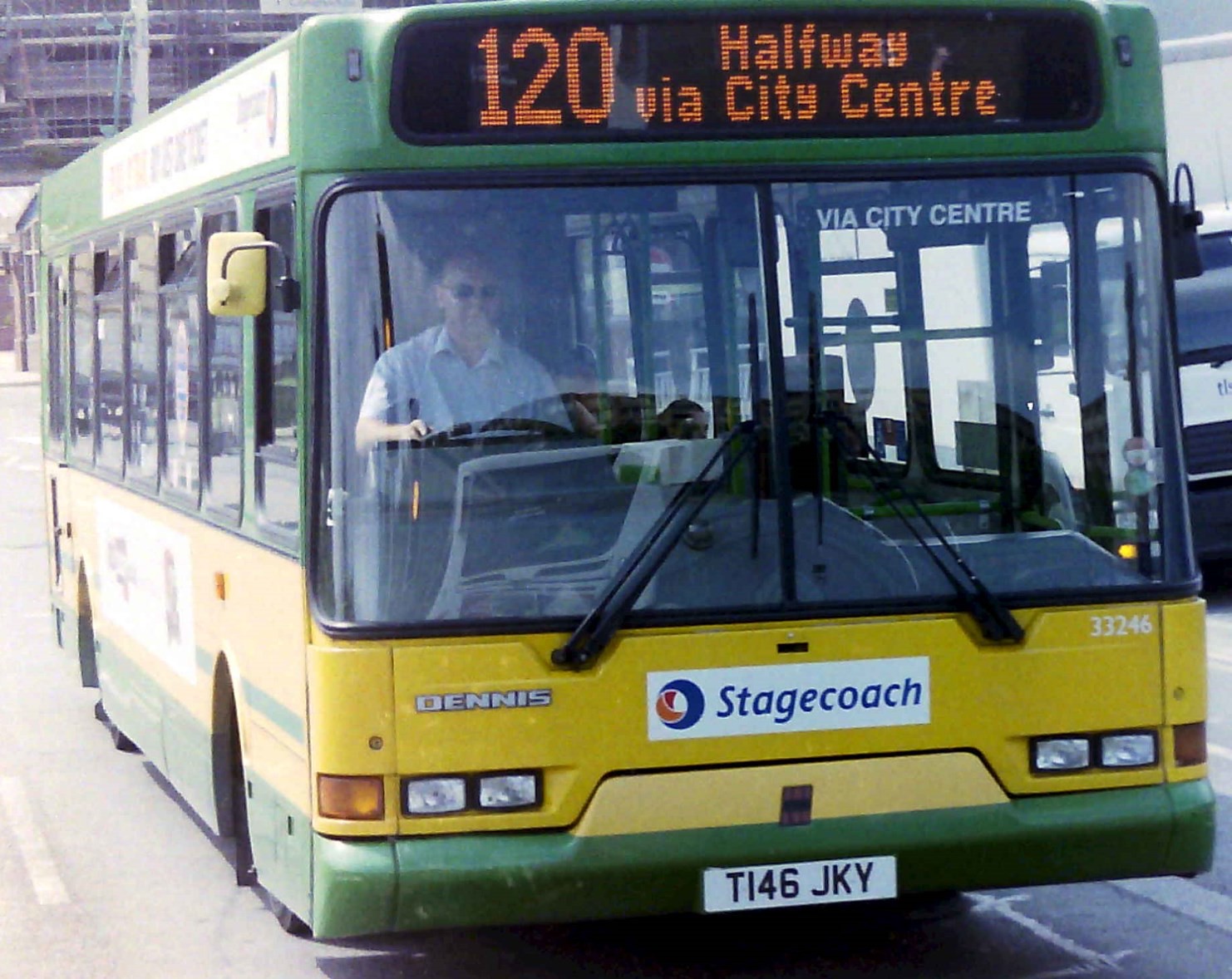In this detailed image, we see a large, yellow and green Stagecoach bus prominently positioned in the center, driving towards us on a typical asphalt road. The bus is captured from a slight diagonal front perspective, showing key details such as the orange LED display reading "120 via Halfway City Center." The driver is visible on the right side, and the bus features the Stagecoach logo on the front. Notably, the bus has a white and black license plate with the name "DENNIS" printed on it. Headlights are situated on both sides of the front grille. The bus appears to be in motion, sharing the road with other vehicles. The surroundings indicate an outdoor setting, likely during the day, with a building visible in the distance. Colors in the image include green, yellow, orange, silver, black, white, and gray, giving a vivid depiction of a city bus navigating through a typical urban landscape.